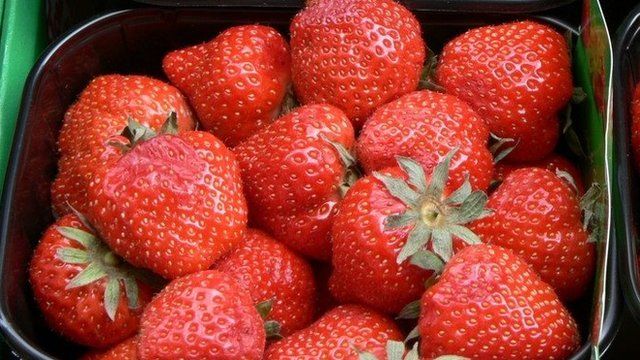The image features a close-up of a centralized, black square bowl filled to the brim with bright red strawberries, taking up nearly the entire frame. The strawberries are fresh and vibrant, each detailed with visible yellow seeds and topped with green leafy stems. They are arranged at various angles, showcasing their ripeness and ready-to-eat appearance. One strawberry on the left side shows signs of beginning to rot with a discoloration to a different pink hue. The image includes no text, focusing solely on the strawberries and the container, which could possibly be plastic or metal. The background is indeterminate, drawing all attention to the strawberries, which dominate the image with their striking red color against the black bowl.